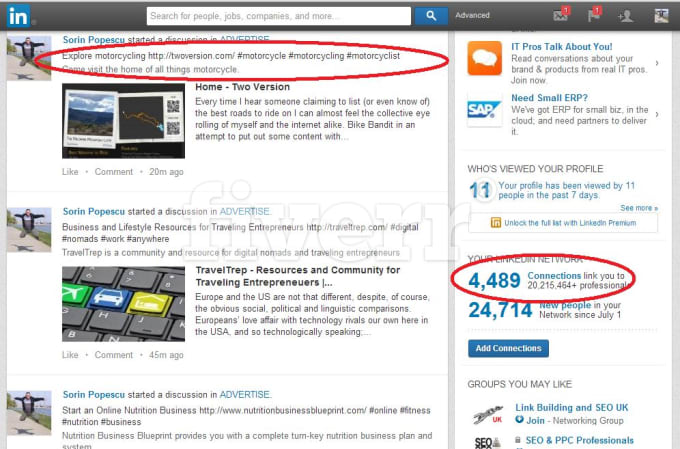**Detailed Caption:**

The image is a screenshot of a LinkedIn interface, recognizable by the prominent white "IN" logo set against a blue background in the top left corner. Adjacent to the logo, a search bar prompts users to "Search for people, jobs, companies, and more." The search button next to it is also blue, followed by an "Advanced" search option. 

On the top right, several icons indicate user interactions: an inbox showing one new message, an icon for friend requests, and the user's profile picture. 

On the left side, a discussion thread initiated by Soren Popescu is highlighted with a red oval. The thread is titled "Explore Motorcycling" and links to toversion.com. Below this, additional details read: "Every time I hear someone claiming to list or even know of the best road to ride on, I can almost feel the collective eye-rolling over myself and on the internet alike."

Further down, two more discussions started by Soren Popescu are featured. The second one discusses "Business and Lifestyle Resources," while the third one focuses on "Starting an Online Nutrition Business."

On the top right, there's a section titled "IT Pros Talk About You," indicating 11 profile viewers in the last 11 days. Beneath this, a statistic displays the user's LinkedIn network with 4,489 connections, linking them to over 20,215,464 professionals, highlighted in red.

At the bottom of the interface, there's a blue button labeled "Add Connection." 

In the center of the image, a faint white watermark reads "Fiverr," subtly marking the origin of the screenshot.